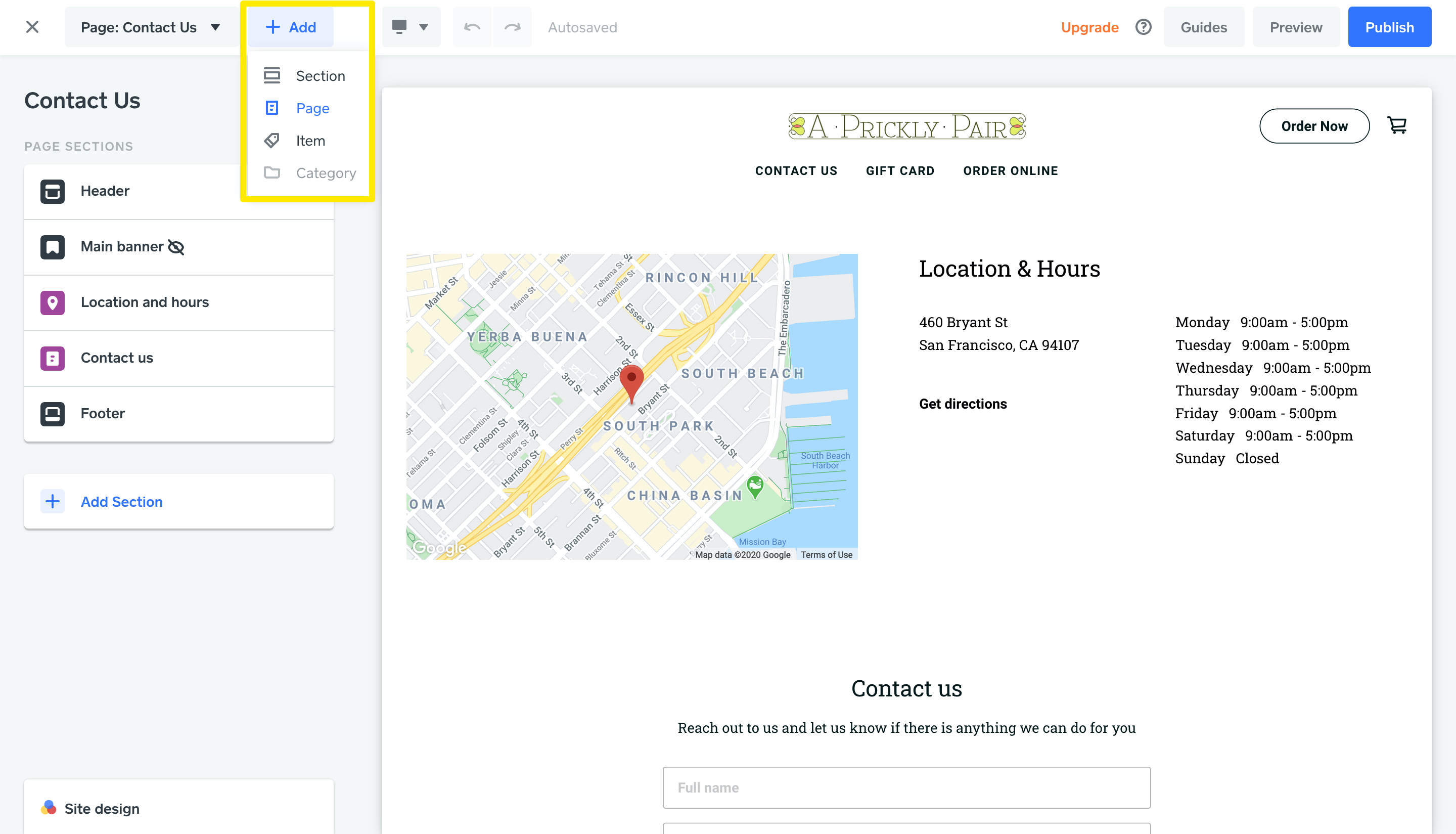This image captures a detailed screenshot of a contact page for a small store named "Prickly Pear," located near South Park in San Francisco, California. Featured prominently is an interactive map highlighting the store's location with a pin. The accompanying text provides the store's address, operational hours (open Monday through Saturday, closed on Sunday), and options to click for directions and contact the store.

Along the left side, a navigation panel lists sections of the contact page: "Contact Us," "Page Sections," "Header," "Main Banner," "Location & Hours," "Contact Us," and "Footer." The contact form encourages visitors to reach out with their name and contact information, emphasizing customer service. However, the image does not specify the products or services offered by "Prickly Pear," which suggests there could be a dedicated section missing from the webpage.